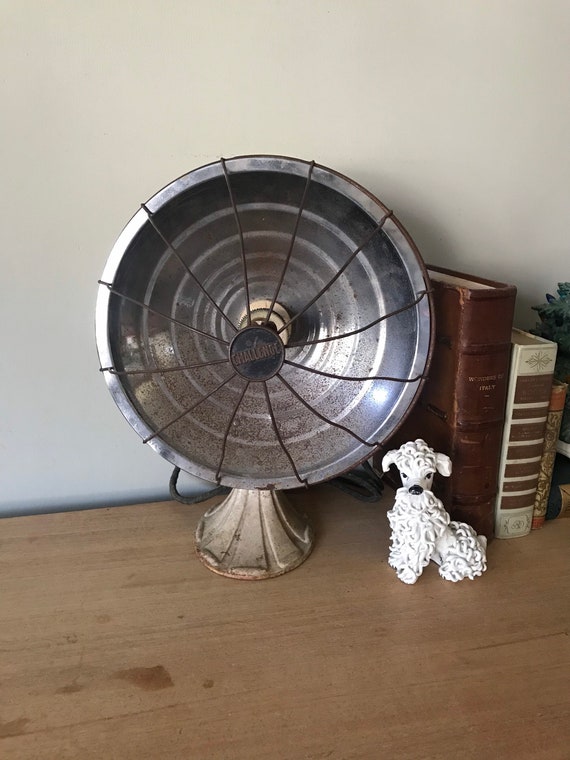In this vertical color photograph, a collection of objects is displayed on a light-colored wooden desk against a white wall. The central object is an old-fashioned parabolic heater with a concave surface and protective metal bars, labeled "Challenge." To the right of the heater is a charming figurine of a white poodle, featuring a black nose and curly black hair. Behind the figurine is a stack of books, including a dark brown book, a white book with brown stripes, a coral-colored book, and a book with a light brown spine. A plant is also visible, adding a touch of greenery to the scene. This detailed arrangement highlights the blend of antique and decorative elements on the desk.